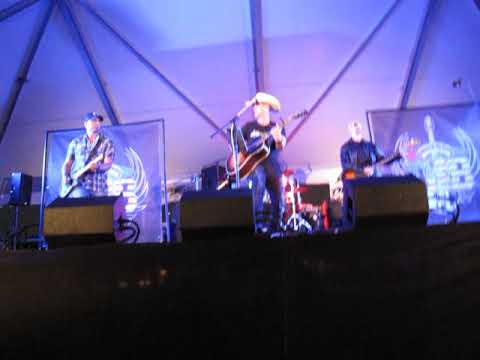The photograph captures a live concert featuring a band performing on stage. The stage is dark, with the bottom third of the image too obscured to discern details. Three main band members are clearly visible. On the left, a man wearing a flannel shirt and a dark-colored hat is playing a guitar. In the middle, the lead singer, dressed in a black t-shirt, blue jeans, and a brown cowboy hat, stands behind a microphone and strums an acoustic brown guitar. On the right, a slightly blurry figure in dark attire, possibly playing a bass guitar, can be seen. All three musicians are Caucasian with rectangular amplifiers at their feet, extending to knee height. The backdrop features two abstract-designed boards or screens, lit by stage lights creating a purple-blue hue. The overall image appears a bit blurry and distant, suggesting it was taken from afar. The concert seems to have a blues rock or country vibe, though the band's identity is not recognizable from the photograph.